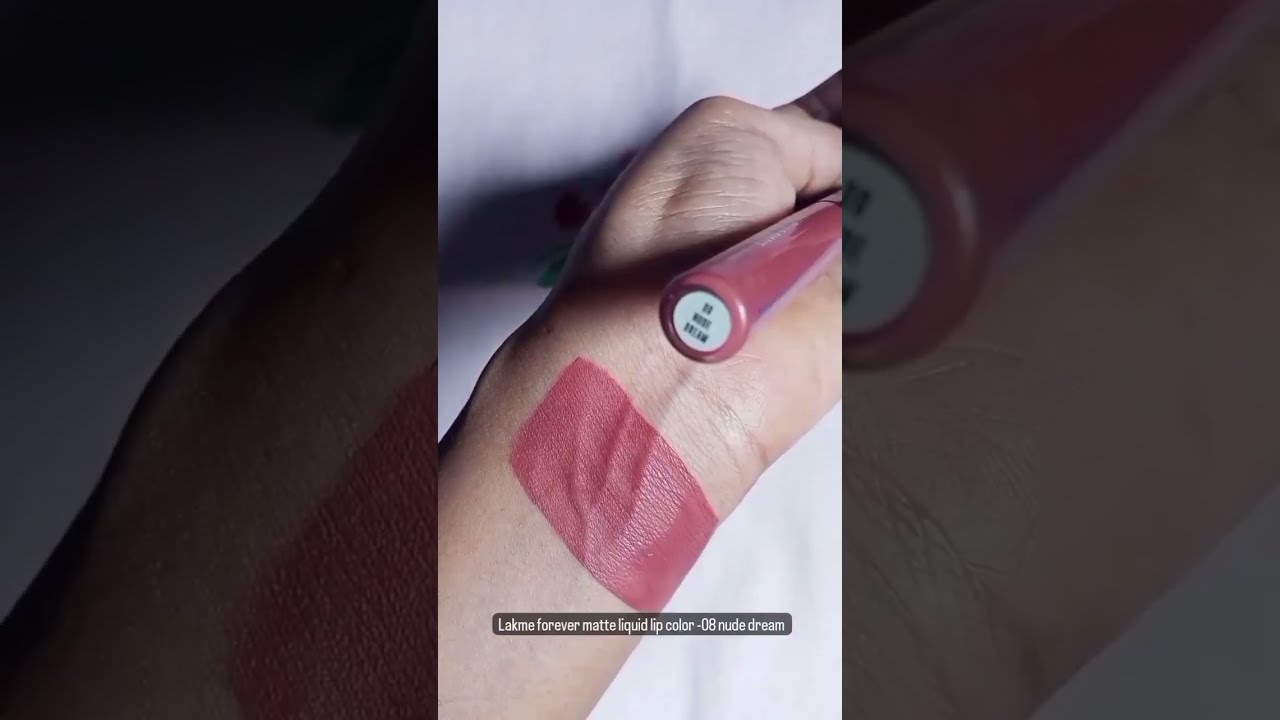The image showcases a detailed close-up of a person's wrist and part of their hand, angled at approximately 45 degrees and centered within a lavender-hued background. The hand grips a tube of Lakme Forever Matte Liquid Lip Color in the shade '08 Nude Dream.' This lip color appears as a rich red, consistent with the swatch drawn in a small rectangle on the person's fair, white European complexion wrist, seemingly to test its appearance against their skin tone. The lip color's cap is a conspicuous white, contrasting with the red liquid. The text, possibly part of a makeup tutorial or review, confirms the product's details. The overall impression suggests the person is documenting the lip color for review or demonstration purposes.